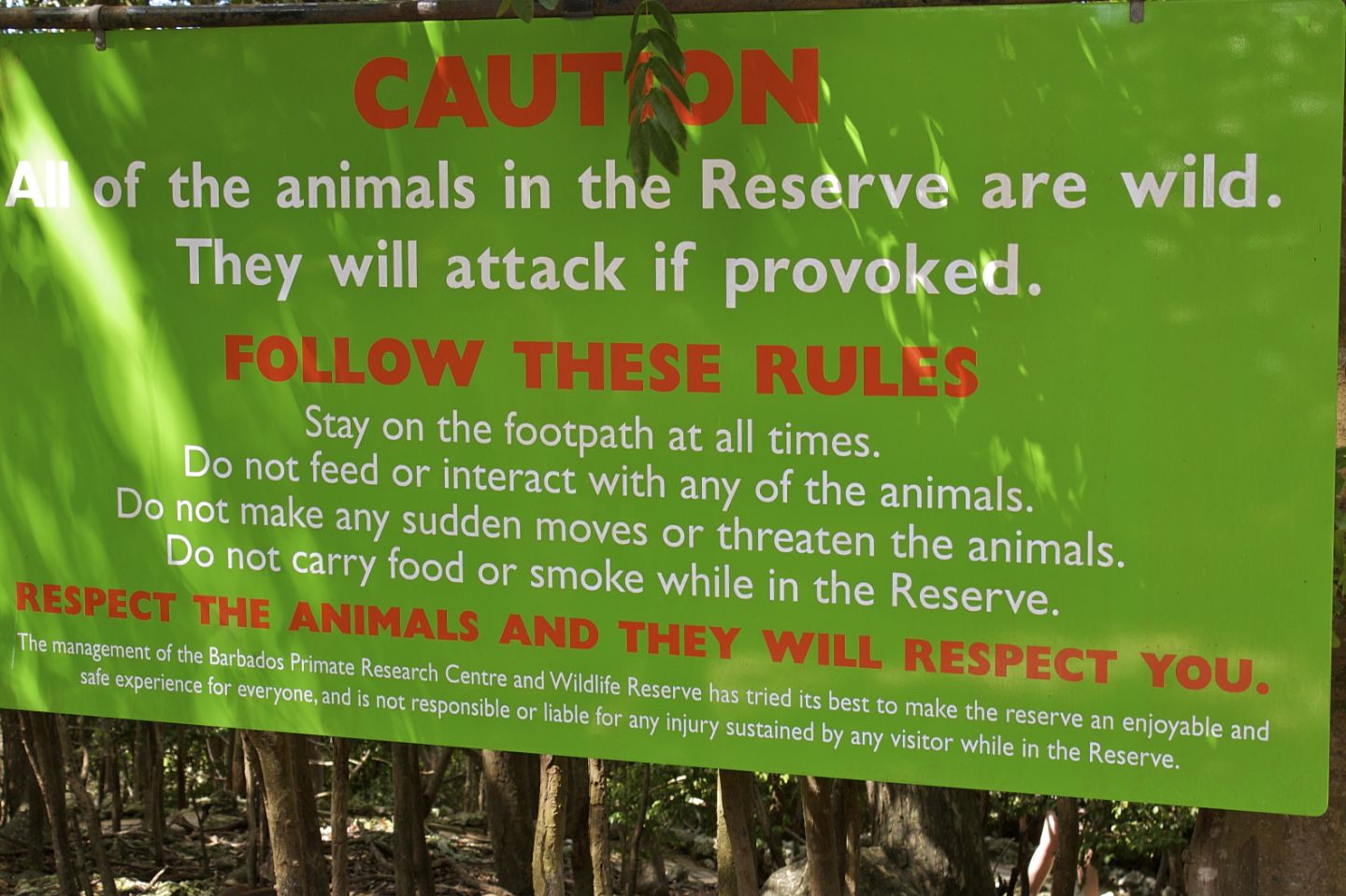The image shows a lime green sign situated in front of a backdrop of trees and plants. The sign features bold uppercase letters in bright orange at the top, stating "CAUTION." Below, in white letters, it warns, "All of the animals in the reserve are wild. They will attack if provoked." The text continues in orange uppercase letters, saying, "FOLLOW THESE RULES." In white, it instructs, "Stay on the footpath at all times. Do not feed or interact with any of the animals. Do not make any sudden moves or threaten the animals. Do not carry food or smoke while in the reserve." Another line in orange reads, "RESPECT THE ANIMALS AND THEY WILL RESPECT YOU." At the bottom, in white letters, it states, "The management of the Barbados Primate Research Center and Wildlife Reserve has tried its best to make the reserve an enjoyable and safe experience for everyone and is not responsible or liable for any injury sustained."